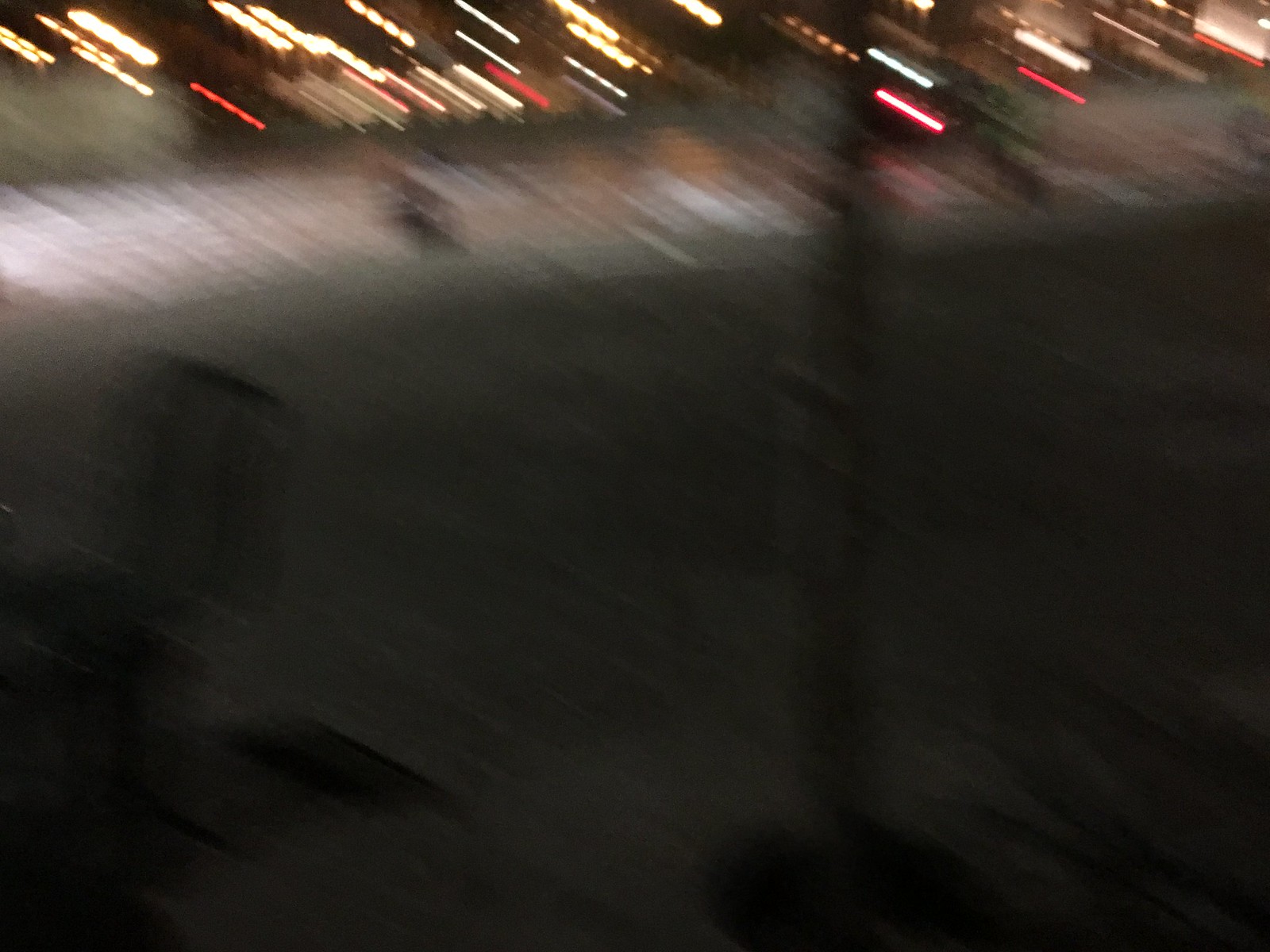A very blurry image predominantly showcases an indiscernible scene with faint details visible. In the upper part of the image, a slanted sidewalk extends from left to right. In the lower left corner, part of a bush is discernible. A thin structure, possibly a tree or a pole, extends from the bottom to the top of the frame, featuring a dark base encircled by a black ring. Faint lights are visible at the top of the image, hinting at an outdoor setting. The overall clarity is poor, making specific identification challenging.